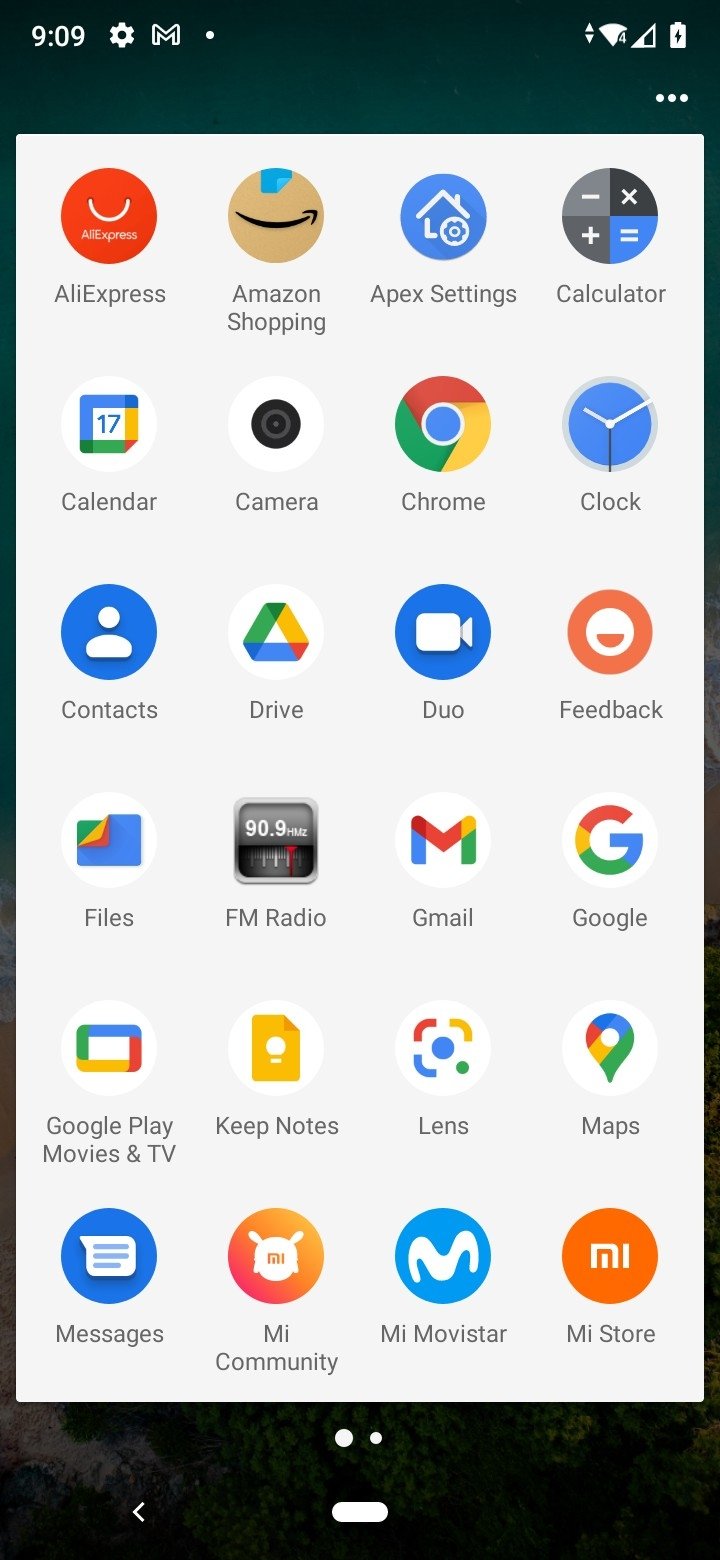Detailed Screenshot Description of a Phone Interface:

This is a screenshot of a smartphone displaying its home screen. The phone features a sleek black trim surrounding the display, with uniform bezels at both the top and bottom. The status bar at the top of the screen shows the time as 09:09, with icons indicating strong internet reception and a fully charged battery. 

The main portion of the screen is filled with a grid of app icons arranged in four columns and six rows, fully occupying the entire view and suggesting that there is no wallpaper image set. 

Here's a detailed list of the icons visible on the home screen, in order:

1. AliExpress - The shopping app icon.
2. Amazon Shopping - Another popular shopping app.
3. Apex Settings - Presumably the settings app for a custom launcher.
4. Google Calculator - The standard Google calculator app.
5. Google Calendar - Google's calendar application.
6. Camera - The phone's camera app.
7. Chrome - Google's web browser.
8. Google Chrome - Appears twice as both the icon and in the search bar.
9. Clock - The app for keeping time, alarms, and timers.
10. Google Contacts - The contacts management app by Google.
11. Google Drive - Cloud storage service icon.
12. Google Duo - Google's video calling app.
13. Feedback - An app, possibly native, unknown to the describer.
14. Files by Google - Google's file management app.
15. FM Radio - Indicates the presence of an FM radio feature.
16. Gmail - The email client by Google.
17. Google - The general Google app for search and news.
18. Google Play Movies & TV - An app for renting and watching movies and TV shows.
19. Google Keep Notes - A note-taking app by Google.
20. Google Lens - Image recognition app by Google.
21. Google Maps - The navigation app.
22. Messages - The SMS and messaging app.
23. My Community MI - Likely an app related to Xiaomi's community platform.
24. My Movie Star MI - Presumably a media-related app by Xiaomi.
25. My Store MI - An app possibly linked to Xiaomi's store or services.

The arrangement and quantity of these apps suggest a highly organized user who prefers using several of Google's ecosystem apps along with popular shopping services and Xiaomi-specific applications.